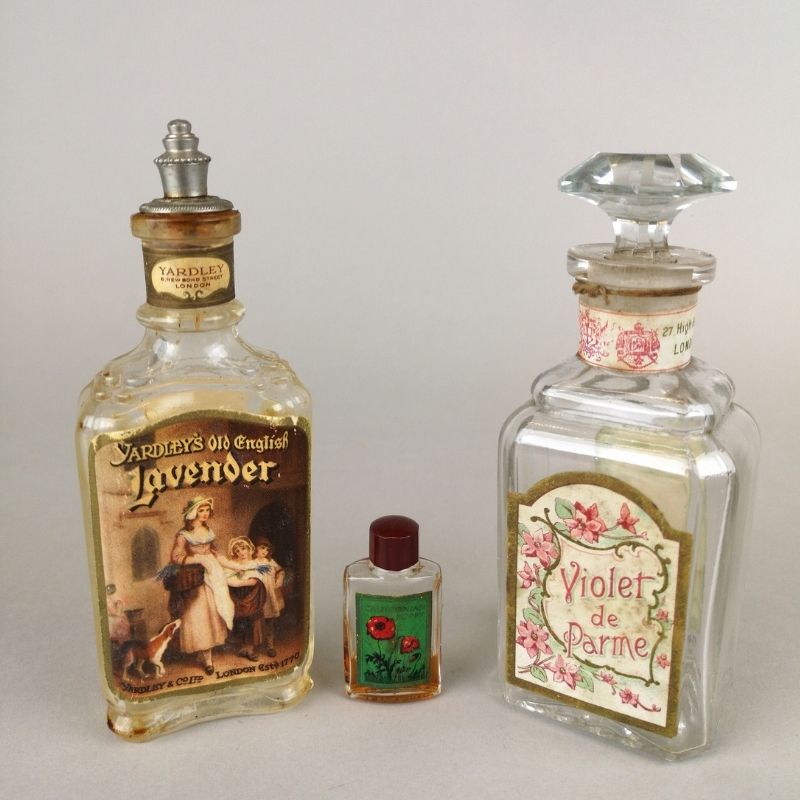The image captures three antique perfume bottles, each with unique characteristics suggestive of their vintage origins, possibly from the Victorian era. The bottle on the left is a clear glass container reminiscent of an old whiskey bottle. It features a tapered neck and is topped with a shiny silver metal cap that includes a cork. The label on this bottle, though worn and stained with age, proudly displays "Yardley's Old English Lavender" in gold text on a brown background. This branding is complemented by a detailed illustration of a woman in a white dress and hat, accompanied by two children and a dog, all standing in front of a building with a window. The label also contains the text "London Estate, 1770."

In the middle stands a much smaller plastic bottle with a dark brown cap. The liquid inside is a rich amber color, and the bottle features a green label adorned with a red rose, though the exact contents and purpose of this bottle remain indeterminate.

On the right is another clear glass bottle, also styled similarly to an antique whiskey bottle. This bottle is cleaner, with no visible stains, and is closed with a diamond-shaped glass stopper. The label reads "Violet De Parma" in a purple-pink font, surrounded by an intricate design of purple-pink roses on green vines against a white background. The neck of the bottle has a similar floral design, matching the elegance and attention to detail seen in the rest of the trio.

These bottles, each with faded labels and signs of aging, contribute to a deeply nostalgic aesthetic, evoking a sense of history and past luxury.